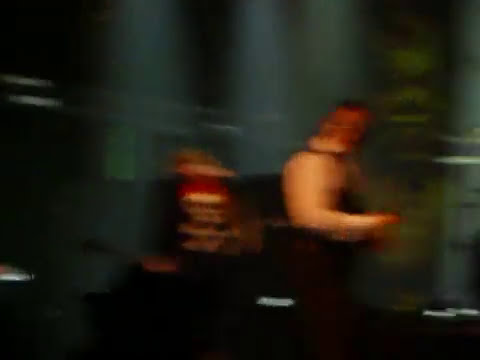The image is extremely blurry with both motion and regular blur, making it difficult to clearly identify the subject. Despite the blurriness, it appears to depict a person standing on a stage or platform, facing right with their head turned towards the left. The person has short black hair and is dressed in a white collared shirt with a black vest or apron. 

Their right arm is visible, extending down with the elbow bent upward, positioning the hand towards the right. Notably, the person has an orange-tinged face, which stands out due to the surrounding darkness. The shirt is a dark black color, and the arm is white. 

In the background, on the left side, various streaks and directional lights are visible. These lights have a cone shape, expanding downward from the top edge of the image, casting shades of white, orange, yellow, brown, and green. The scene is set in a dark room with numerous lights and some darker shadows. Towards the right, there is a large, indistinct stacked object made up of tans, whites, and reds, which is difficult to identify due to the blur. The bottom of the image features the silhouette of a raised black countertop, framing the scene.